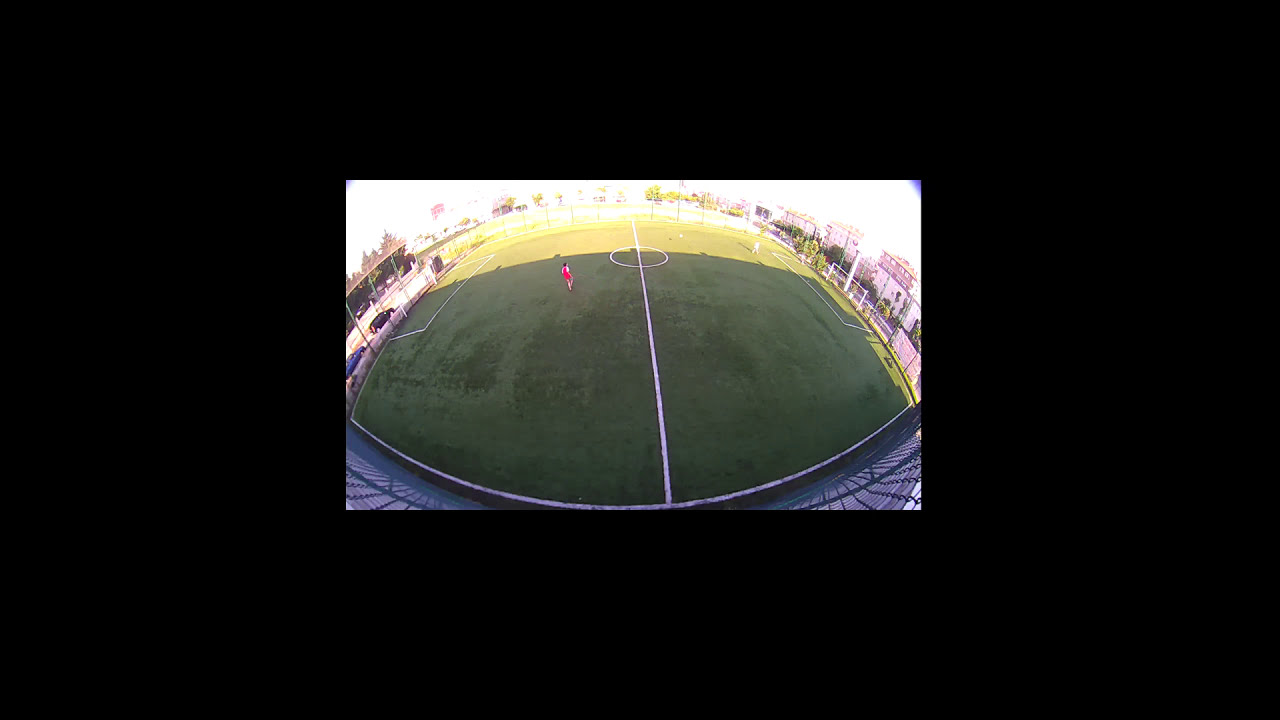This detailed aerial photo of a soccer field captures the lush green turf divided by a white center stripe and a distinctive white center circle. The field is bordered by white rectangular goal lines on both ends. The sunlight brightens the left half of the field, casting it in a light green glow, while the right half appears a darker green due to the shade. The field is fenced around its perimeter, with parked cars visible on one side. The overcast, hazy sky contributes to the muted lighting conditions, giving the day a white, clouded appearance. On the field, two players can be seen: one in a red jersey and another in a white jersey, engaging in the game. Additional people are spotted in the upper right corner of the image. The perspective, framed by black rectangles, suggests a 360-degree view, creating a slightly warped appearance that elongates the field visually.